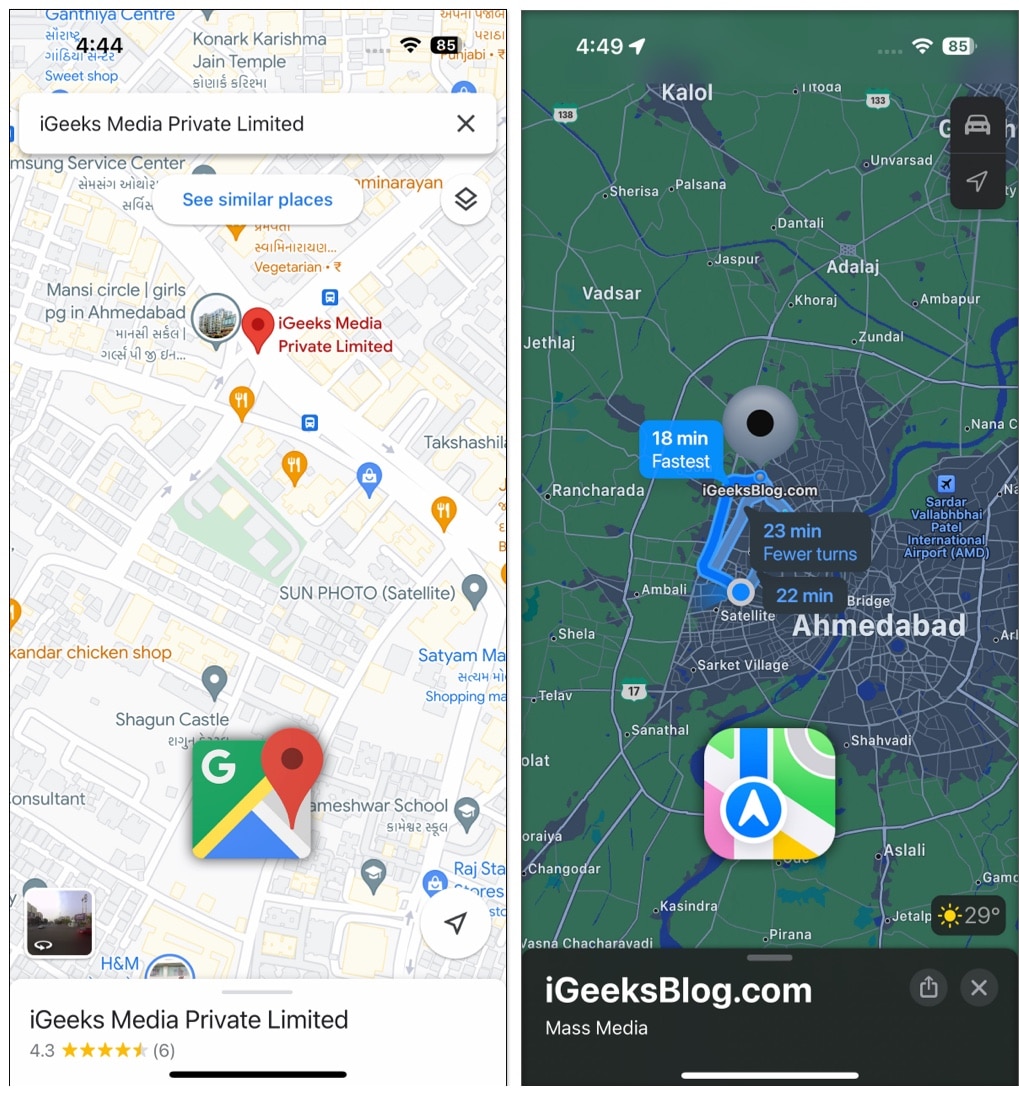This post features two side-by-side screenshots comparing map views from different search engines. The screenshot on the right is from iGeeksBlog.com, displaying a broad map view with green landmasses, blue waterways, and city buildings marked in dark gray. This map seems to be more generalized, potentially using Apple's search engine. In contrast, the left screenshot, likely from Google Maps, provides a detailed, zoomed-in view of the specific location of iGeeksMediaPrivateNetwork. The Google Maps view showcases streets and buildings with greater clarity, making it easier to pinpoint the company's exact location. The distinctive "G" logo in the top corner indicates the use of Google's search engine, facilitating a more focused and detailed representation of the area.